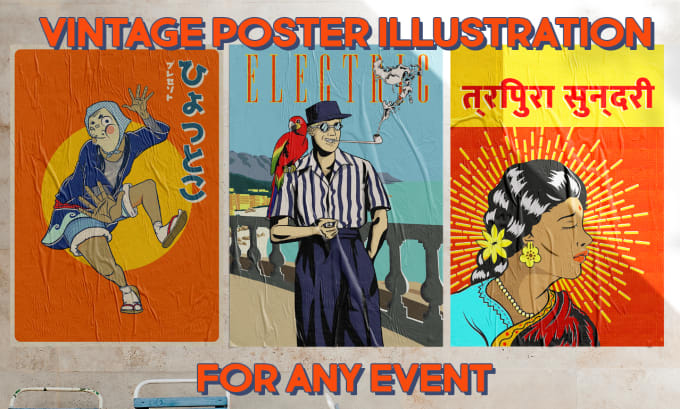An advertisement image for vintage poster illustrations prominently showcases three distinct illustrated posters set against a white wall and framed by a vibrant orange border. The top of the image reads "Vintage Poster Illustration for Any Event." 

The poster on the left, featuring Japanese text, displays a man in mid-jump wearing a blue coat, shorts, flip-flops with socks, and framed by a yellow sunburst in the background. The background is a bold orange-red, adding to the poster’s energetic feel.

The center poster, with a light blue background, depicts a man standing in front of a stone fence overlooking the ocean. He is dressed in a black hat, a black and white vertically striped shirt, and black pants. A red parakeet perches on his right shoulder, and he is blowing smoke from a pipe. The word "Electric" is prominently featured on this poster.

The right-hand poster, depicting an Indian theme, has a gradient background transitioning from yellow at the top to orange at the bottom. This poster highlights a profile view of a woman with tan skin, closed eyes, black hair streaked with white, and adorned with a yellow flower and sunshine-like rays behind her head. She is wearing a blue sari and a pearl necklace. There are also illegible Middle Eastern-like characters at the top of the poster.